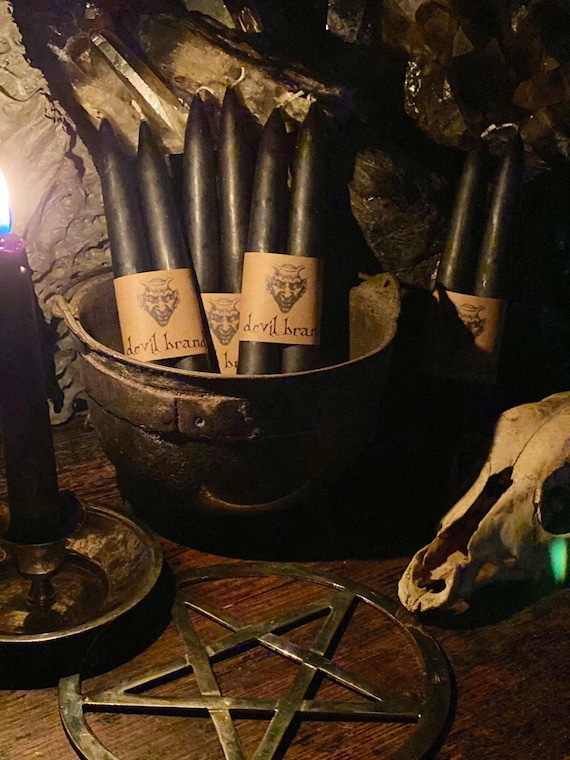In this indoor image, likely set inside of a cave, the scene is dark and atmospheric, shifting towards a gothic or possibly satanic theme. The background reveals a craggy stone wall, providing a rugged and eerie ambiance. Dominating the foreground is a dark wooden table, rich with varying hues of brown. On the table lies a weathered bronze pentagram, boldly etched within a circular metal disk. To the left of this star, there is a stark white cattle skull, adding to the macabre setting.

Centrally positioned on the table is an old, rusted bucket filled with three pairs of black, tapered candles. These candles are bundled together with brown paper bands, each adorned with a devil's face and labeled "Devil Brand." Another similar set of loose candles rests against the stone wall. On the left side of the table, a candle holder supports a lit red candle, its flame flickering and melting wax running down its side, casting an eerie glow over the scene. The overall photograph leans towards a portrait orientation, capturing the dark, mystical, and ritualistic atmosphere in striking detail.